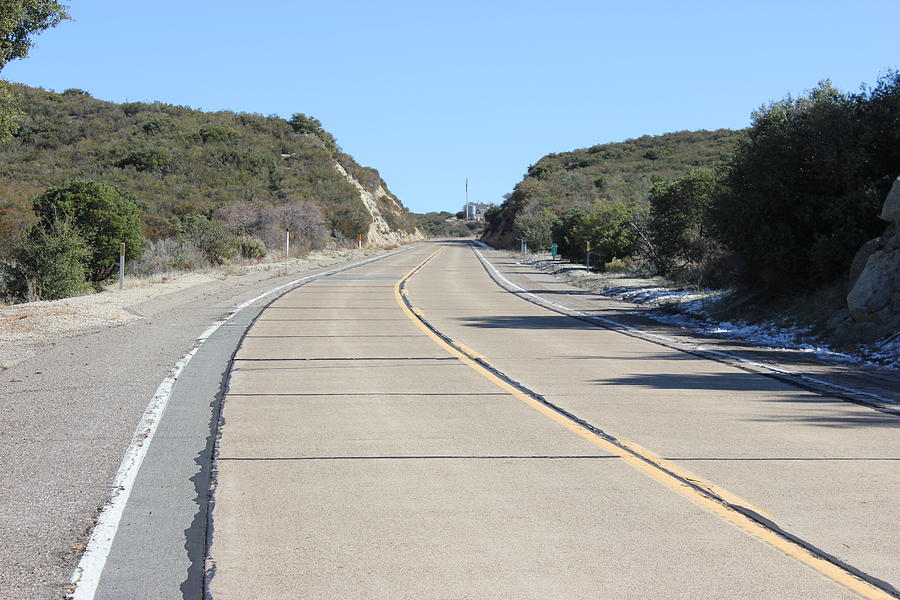This professional-quality photograph captures a serene scene of an empty two-lane road winding through a lush, mountainous landscape. The road, made of concrete, features a primary double yellow line down its center, accompanied by dotted yellow lines and flanked by solid white lines on either side. Adjacent to the road are green bushes and trees resembling clusters of broccoli florets, interspersed with patches of brown, dying foliage. The road's edges are lined with gravel and notable features like white rocks and a green box attached to a pole. Additional details include mile markers scattered along the left side of the road and a distant view of a mountain straight ahead. Overhead, the sky is a flawless, even blue, marking a clear, sunlit day. The colors in the image are kept simple yet vibrant, featuring black, white, gray, yellow, blue, and green hues. The scene is devoid of people, animals, and buildings, except for a possible distant structure with an American flag and a water tank, making it feel peaceful and isolated.